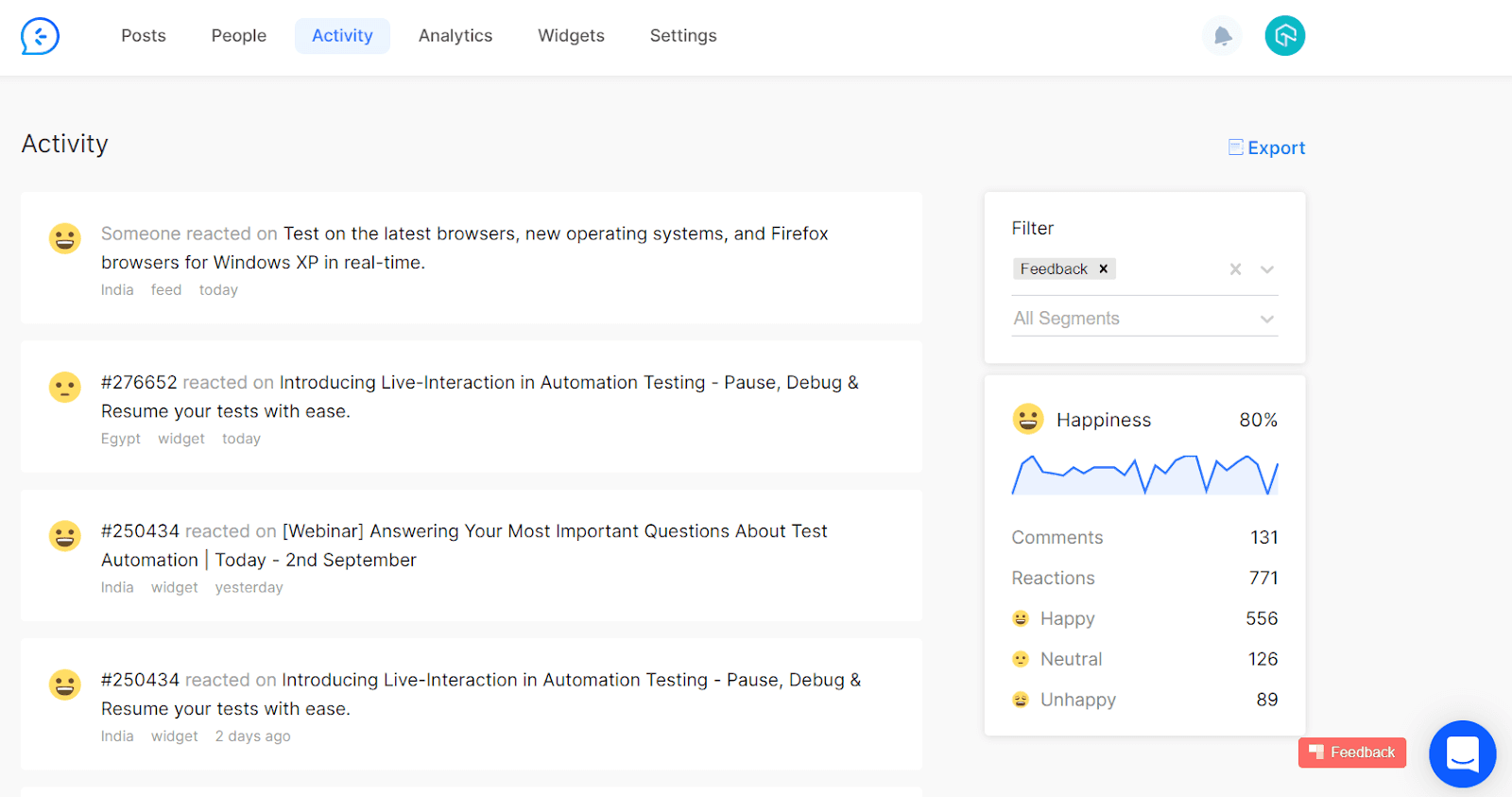A vibrant activity page from an unidentified website featuring a logo. The top navigation bar includes tabs for Posts, People, Activity, Analytics, Widgets, and Settings, with the Activity tab currently highlighted. Detailed real-time updates populate beneath the Activity label, indicating user interactions such as:

- A user reacting to a post about testing new and existing browsers, including Firefox for Windows XP.
- User activity under entry number 276652, which involves reactions to the introduction of live interaction and automation testing, highlighting features for pausing, debugging, and resuming tests with ease.
- The presence of a potentially significant entry responding to questions about test automation.
- Repeated emphasis on new functionalities for live interaction and automated testing, enhancing user test management capabilities.

To the right, a prominently displayed chart, labeled as the "happiness chart," visually suggests a satisfaction level indexed at 80%. The page might be part of a bug tracking or learning platform, focused on software testing and automation, though the exact nature remains unspecified due to the lack of clear contextual information.